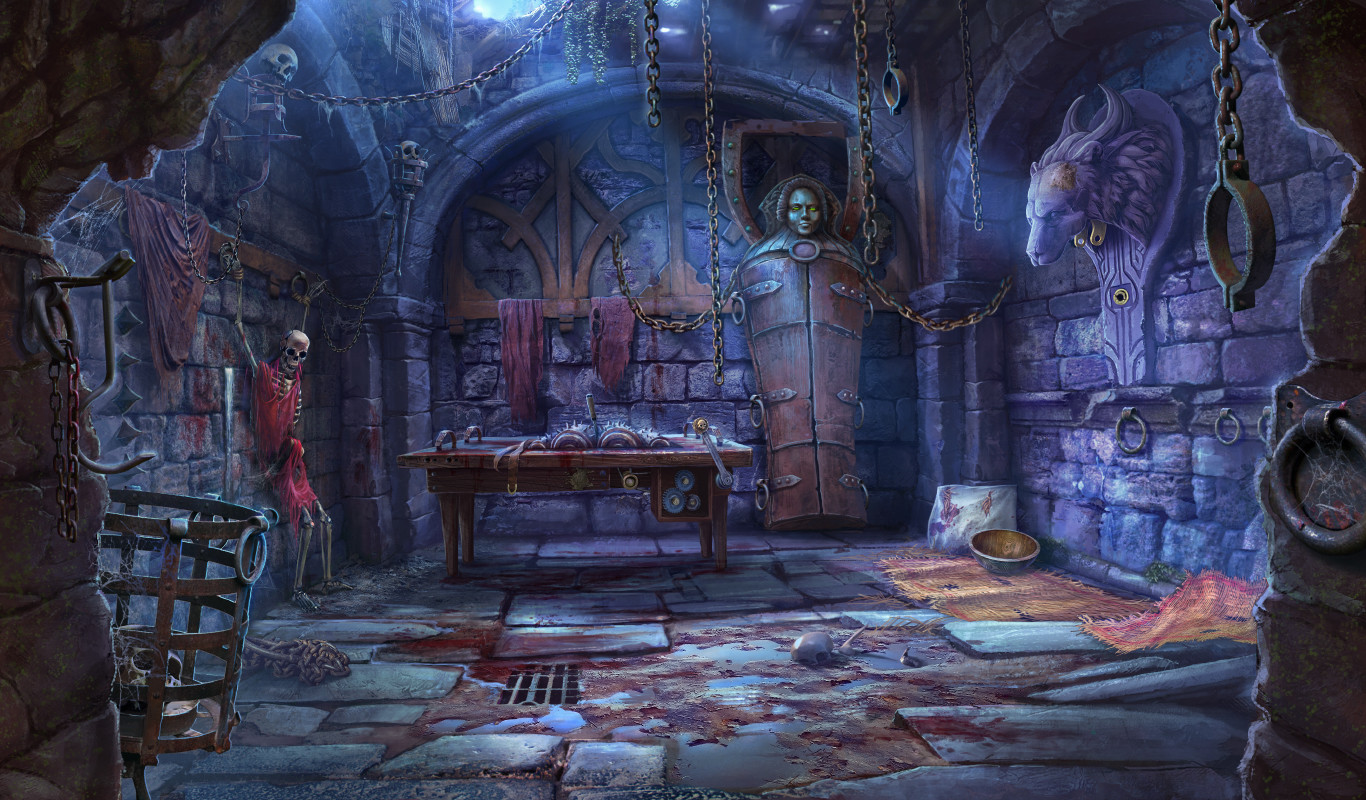The animated picture depicts a gruesome dungeon bathed in a purplish-blue hue, with sunlight filtering through a small, high window. The stone walls are cracked and etched with various symbols, enhancing the eerie, ancient atmosphere. To the left, a skeleton in a red tunic is shackled to the wall, symbolizing the horrors endured within this dungeon. Bloodstains mar the rock floor, evidence of past violence and terror. The right wall features a mounted animal head, likely from a horned creature like a water buffalo, adding to the macabre decor. Chains and cages hang ominously from the ceiling, reinforcing the scene’s grim purpose as a torture chamber. Towards the back, a large wooden table, stained with the history of prisoners and unspeakable acts, stands in front of an upright casket-like structure with a grotesquely oversized, monstrous human head protruding from it. This nightmarish tableau suggests a place where atrocities were once commonplace, evoking a sense of dread and desolation.